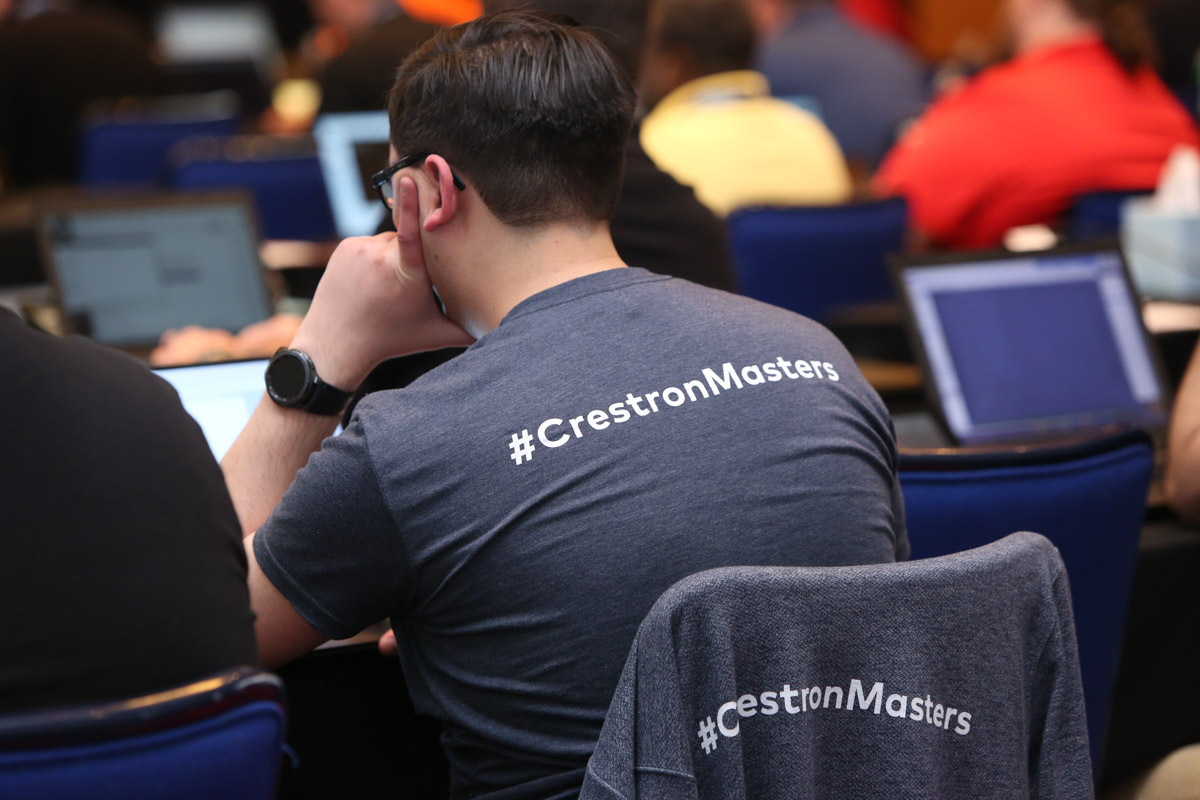In this detailed photograph, the focal point is the back of a man seated at a table, surrounded by rows of other individuals who are all engrossed in their laptops. The man, clearly the main subject, wears a Heather gray t-shirt with the inscription "#CrestonMasters" in white on the back. Draped over the back of his chair is a matching gray sweater, also emblazoned with "#CrestonMasters." He has short, dark brown hair and is wearing black glasses. His head rests on his left hand, showcasing a large black watch on his wrist. The setting appears to be a lecture hall or classroom, suggested by the numerous blurred figures similarly positioned at tables with open laptops. The seats are predominantly blue, and the background features a variety of colorful t-shirts worn by the other participants.